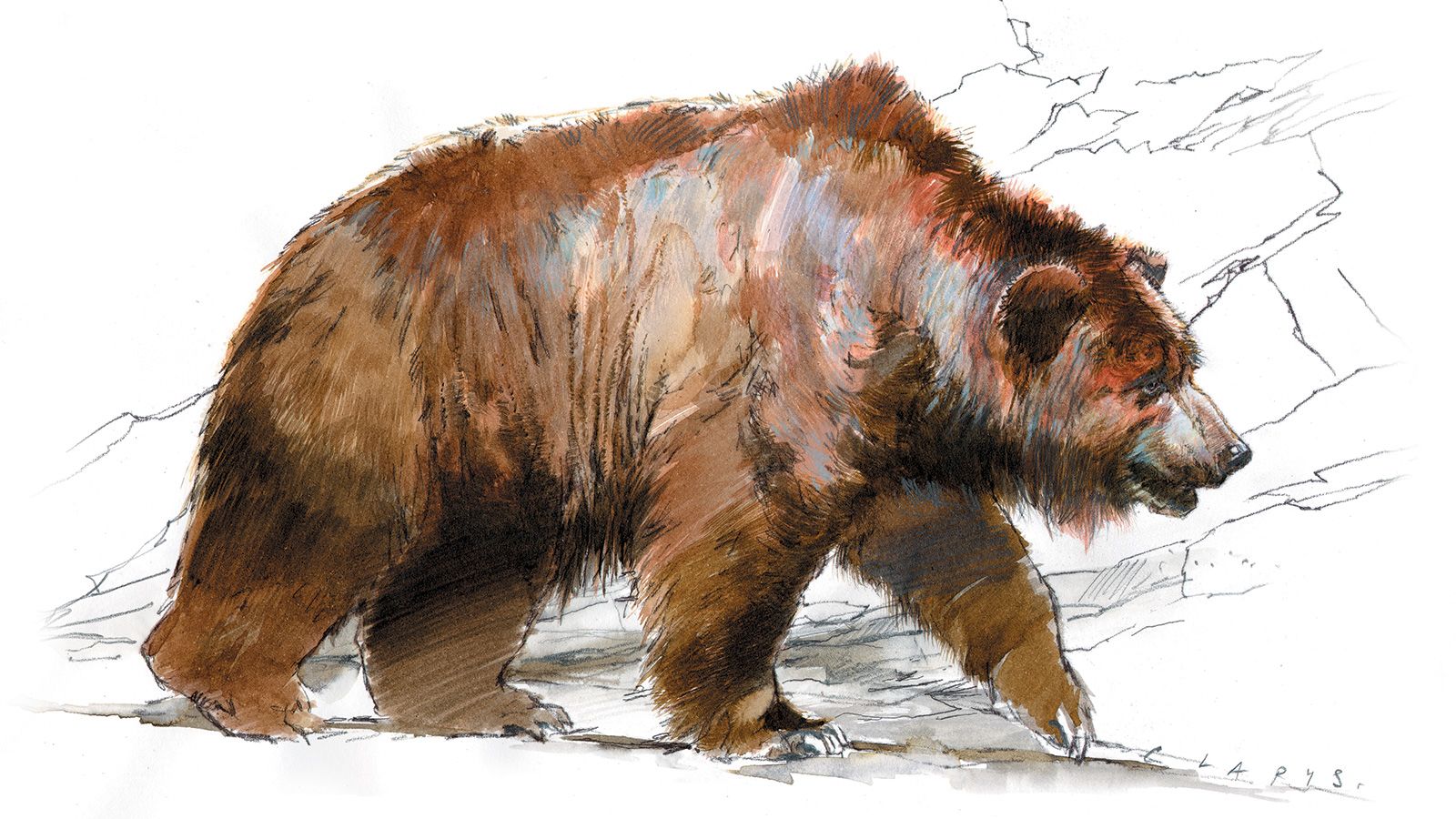This is a finely detailed digital drawing resembling a traditional artwork, depicting a large brown bear with rich textures and well-illustrated shading. The bear's fur showcases a blend of browns, tans, reddish-browns, and hints of gray, capturing the hair's depth and texture. The majestic creature appears to be trudging along, perhaps on a hillside or through a forest, with a weighty presence that suggests it could be around 300 or 400 pounds. In the background, a series of uncolored black line-drawn mountains add a stark contrast to the bear, emphasizing its solitude and natural habitat. To the bottom right, the name 'Calypso,' presumably the artist, is inscribed. Despite the limited color palette, the intricate detailing and realistic portrayal convey a vivid scene of the bear in its environment.